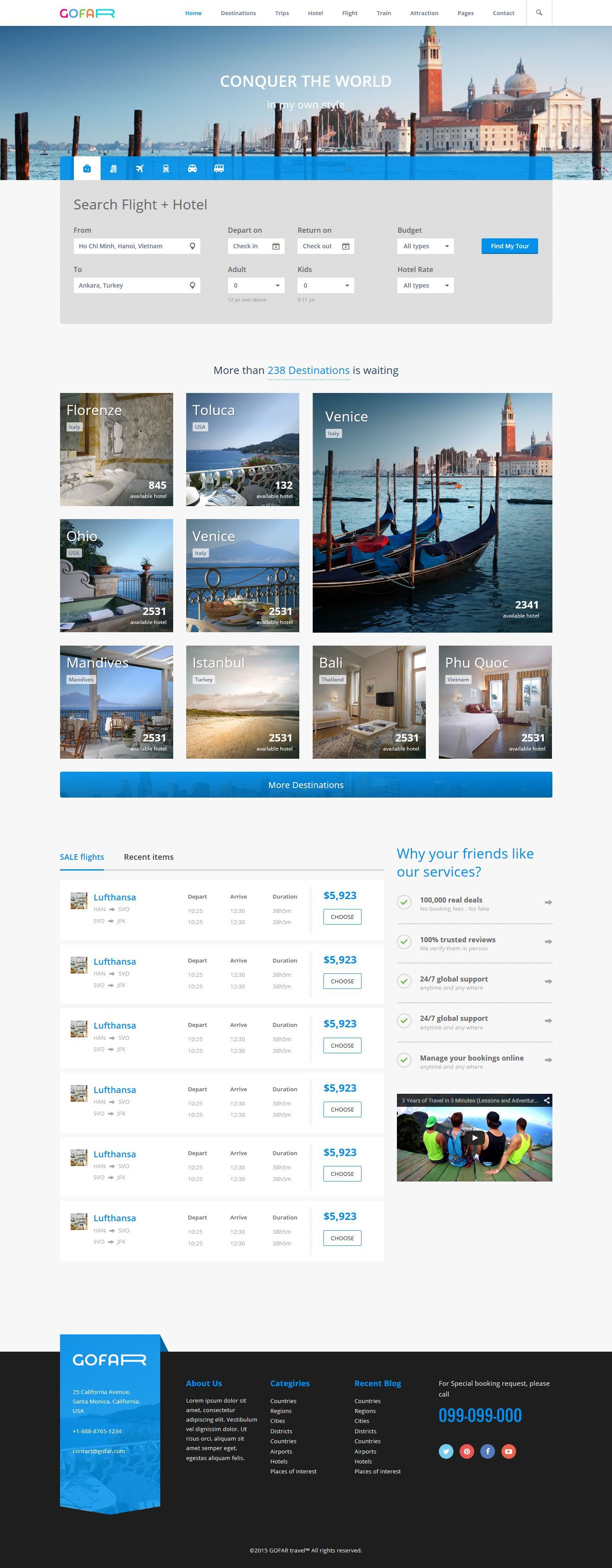The image is a comprehensive long screenshot capturing the entirety of a website's homepage. The top banner prominently features an inspirational slogan, "Conquer the World," set against a visually striking background image of a bustling cityscape, imbuing a sense of global exploration and adventure. 

Beneath this tagline, the website presents a user-friendly section dedicated to searching for flights and hotels. This section is equipped with a variety of dropdown menus and input fields allowing users to fine-tune their travel options. Choices such as destinations, dates, and passenger details can be selected from these menus, providing a streamlined booking experience.

Following the booking section, the homepage showcases an array of enticing thumbnails, each representing different travel destinations. Prominent among these are vibrant images of Bali, with its lush greenery and serene beaches; Venice, with its iconic waterways and picturesque architecture; and Malaysia, with its dynamic blend of modern skylines and cultural landmarks. Each destination is accompanied by its respective price listing, offering potential travelers a clear idea of the cost associated with visiting these locales.

Overall, the detailed layout and inviting imagery of this homepage effectively cater to the wanderlust of users, encouraging them to explore and plan their next adventure.